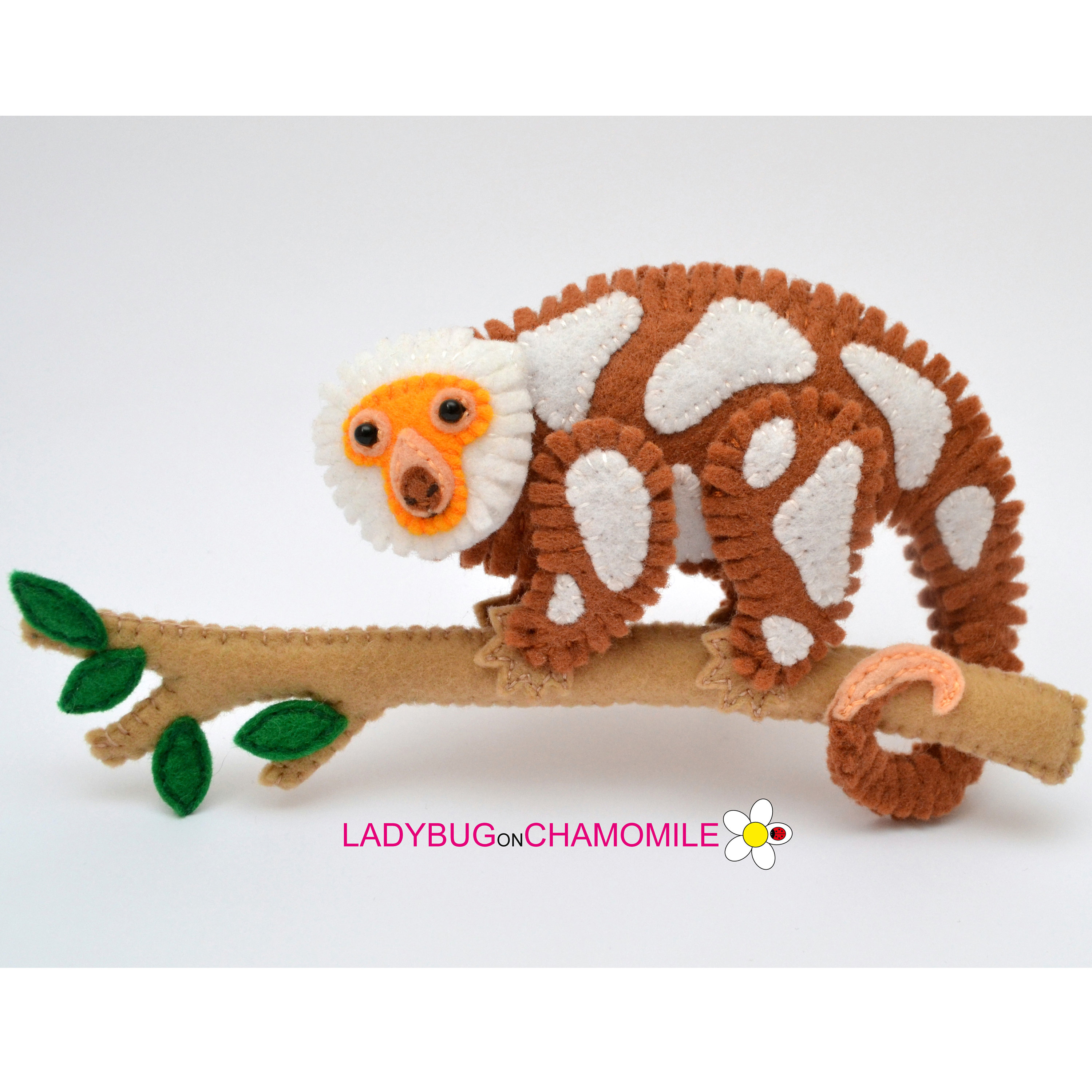In this image, we see a handcrafted felt lemur with a body that features a brown base with white splotches and an orange face. The lemur is detailed with sewn-on eyes and a nose, which is a combination of pink and brown. He is clinging to a tan felt branch adorned with four green leaves towards the left side, and his tail is wrapped around the back of the branch. The background is a light gray, providing a neutral backdrop that emphasizes the main elements. Below the lemur and the branch, the text reads "Ladybug on Chamomile" with 'Ladybug' and 'Chamomile' written in pinkish-purple letters and 'on' in smaller black letters. Adjacent to this text is a small daisy flower logo featuring a ladybug. The primary colors in the image are brown, white, orange, tan, green, pink, and gray. The overall aesthetic suggests a meticulously crafted project intended for display or sale.